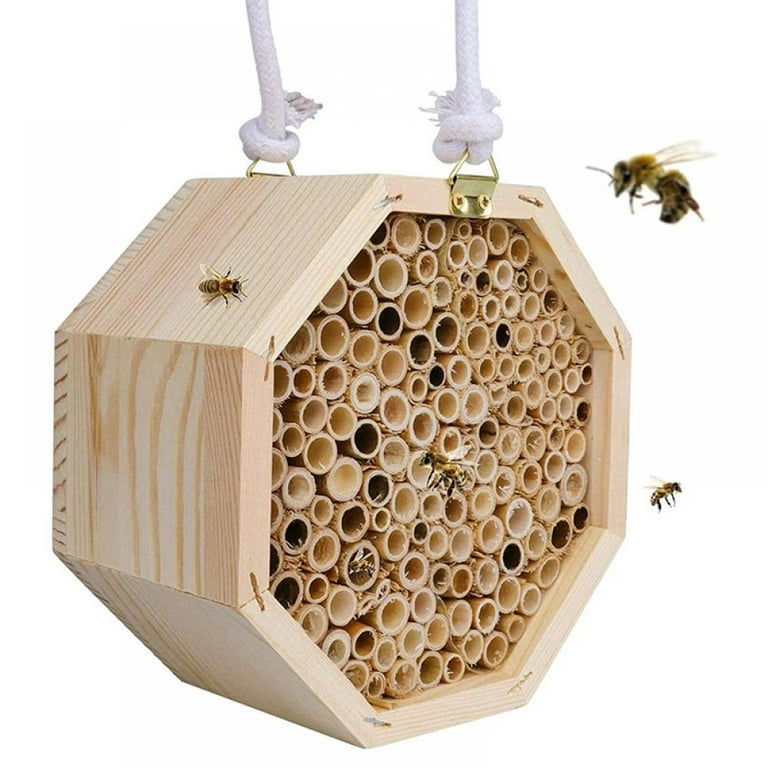The photograph depicts an up-close view of a homemade wooden beehive, crafted in an octagonal shape with a honeycomb-like design. The structure consists of multiple round, hollow wooden compartments where honey bees are actively working. Some of these tubes are occupied by bees depositing wax and generating honey, while others remain empty. The wood is a clean-cut, pale oak, giving it a natural, unvarnished appearance. The hive is suspended by two thick white nylon ropes attached to brass fittings, suggesting it is designed to hang. Approximately ten honey bees can be seen flying around the hive, one bee is prominently entering a tube, and another is crawling along the left side. The background is a white void, making the beehive the central focus of the image, which suggests it might be featured in a store product page.